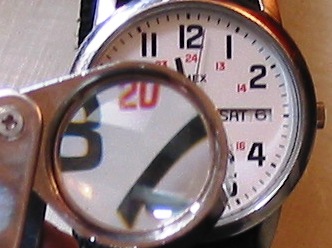In the foreground of the image, there's a silver magnifying loupe, known as a triplet lens, strategically positioned over a wristwatch to provide a closer look at the watch's face. The loupe is designed with a metal cover that can be folded to protect the lens when not in use, and extended when needed for magnification. It is placed over the 7 and 8 o'clock region of the watch's dial, significantly enlarging the view of the minute hand and the small red number 20, which corresponds to the 8 o'clock mark on the 24-hour clock.

The watch itself, occupying the background, is strapped to what is presumably someone's wrist; we can see the edges of their flesh flanking the watch. The watch has a classic circular face, with its top and bottom edges touching the boundaries of the image. The watch face is white, adorned with bold black numbers indicating the hours from 1 to 12. Positioned below each black hour numeral are smaller red numbers ranging from 13 to 24, which represent the PM hours on a 24-hour clock.

On the right side of the watch's face, there is a wind-up knob, establishing that it is a mechanical watch. Between the 2 and 4 o'clock positions, a small rectangular slot displays the day of the week and date, currently showing "Saturday 6." The detailed and precise structure of the watch, coupled with the magnifying loupe, underscores the intricacy and craftsmanship involved in such timepieces.